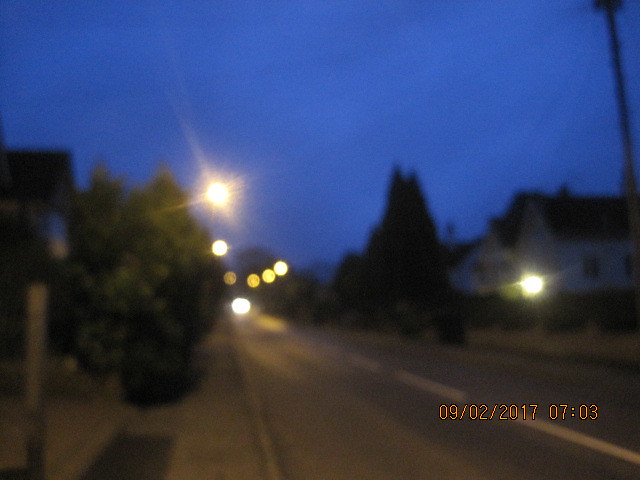The surveillance footage dated 09.02.2017 at 07:03, displayed in yellow text at the bottom, captures a blurry and out-of-focus street scene during what appears to be early morning. The scene is set in a small town residential area with a dark blue sky overhead. The focal point includes a wide two-lane road lined with tall shrubs, possibly evergreen trees, and dotted with six street lamps casting blurry lights. Among the elements of the image, a white house stands out on the center-right, with a bright light illuminated near its doorway. Blurred headlights from a distant vehicle suggest activity, enhancing the tranquil yet fuzzy early morning ambiance. Additionally, there is a noticeable sidewalk on both sides of the street and what seems to be a boxy building, potentially an apartment or business, vaguely visible on the left.